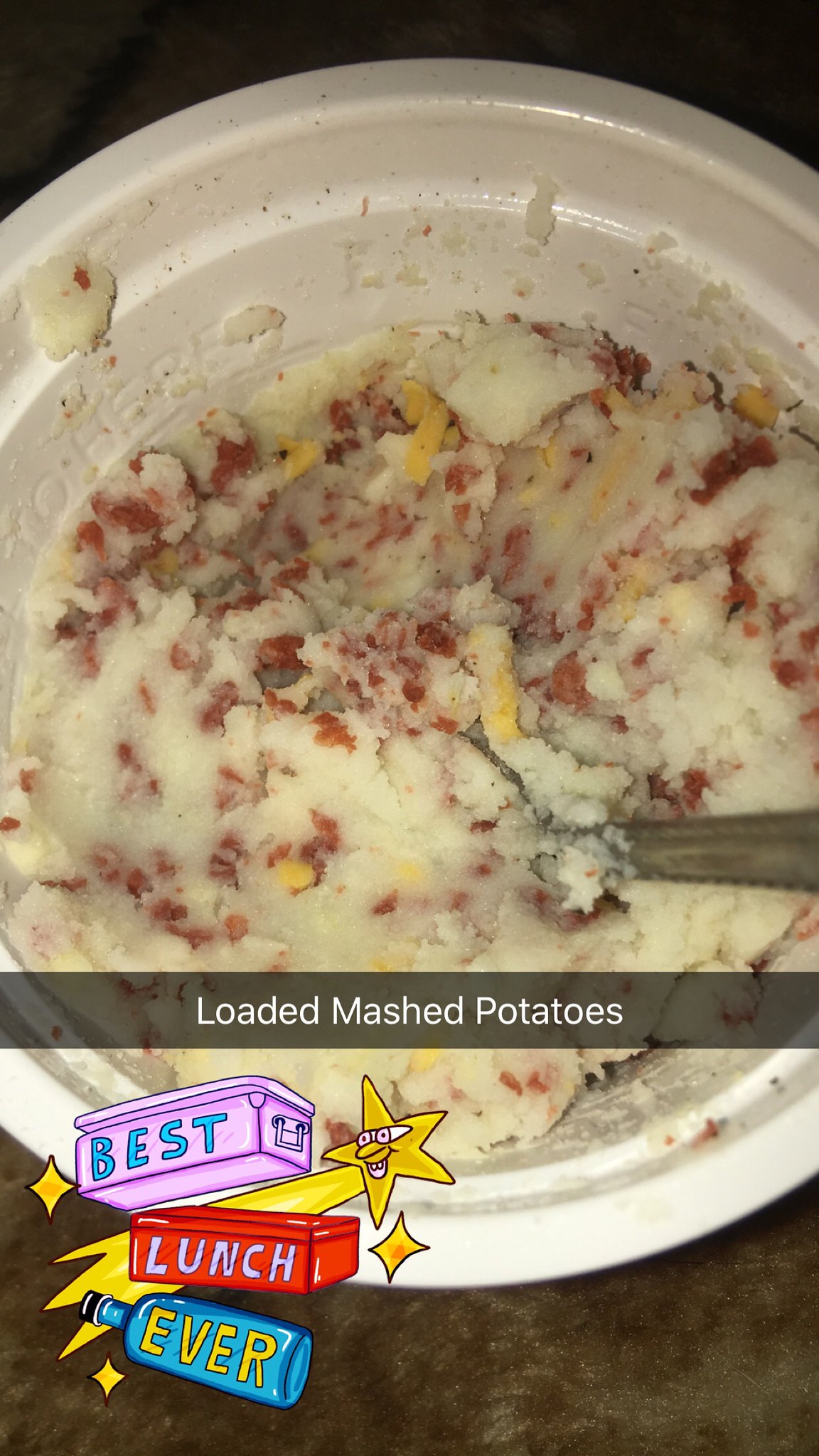The image is a top-down photograph of a large white styrofoam bowl filled with loaded mashed potatoes, positioned on a tan table. These potatoes are mixed with chunky bacon bits, shredded cheddar cheese, and possibly some red spices. A silver spoon is partially visible, stuck into the mashed potatoes, though the tip extends beyond the top edge of the photo. A translucent gray banner spans the lower part of the bowl, displaying the text "loaded mashed potatoes" in white lettering. In the lower left-hand corner of the image, there is a whimsical graphic with two food containers and a bottle on its side. The top container is pink with the word "best" in blue letters, the middle container is red with "lunch" written in lavender letters, and the blue bottle lying horizontally bears the word "ever" in yellow letters. Surrounding this graphic are three yellow diamonds and a cheery yellow star with a white face, enhancing the playful, cartoon-like theme of the design.